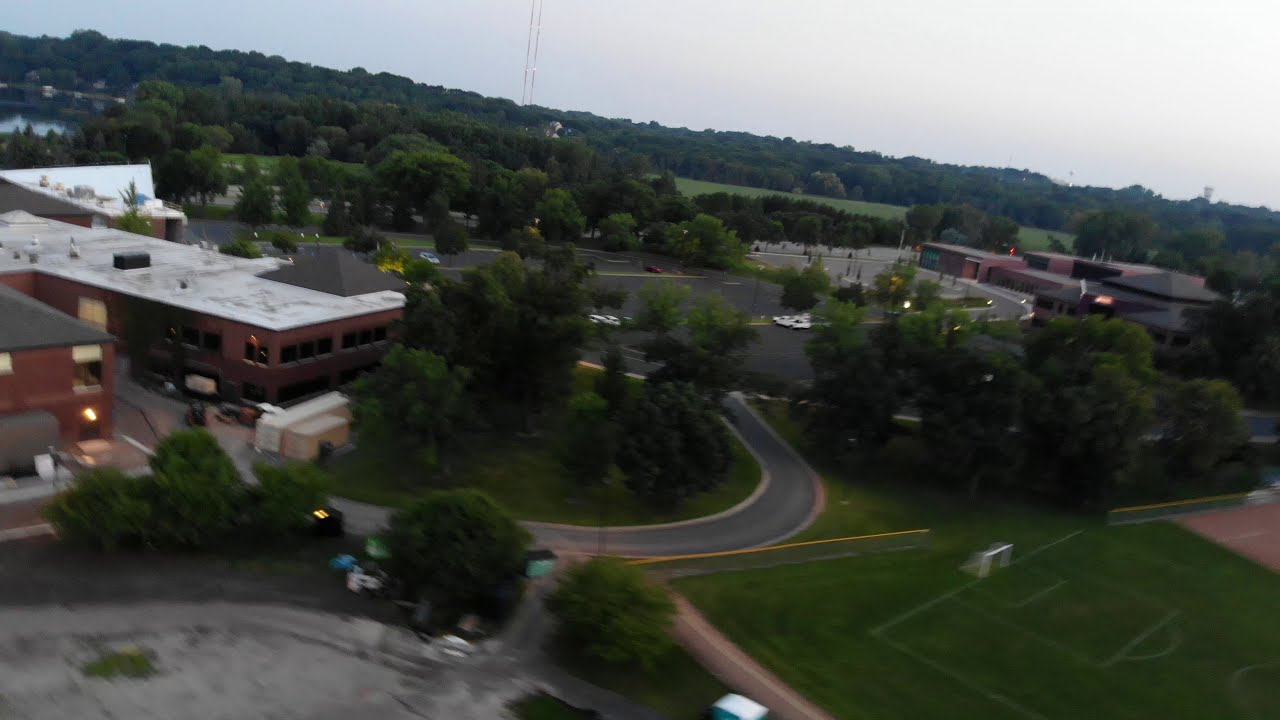This image depicts a somewhat blurry and tilted view of a possible school complex surrounded by nature. Dominating the left side is a red brick building with a flat white roof featuring several gray peaks and multiple windows. This structure appears to be a couple of floors tall. Just in front of this building lies an expansive, relatively empty parking lot with a few cars scattered throughout. A road emerges from the bottom of the parking lot, curving to the left and leading up to the brick building. To the right side of the image, another structure, likely part of the same school, can be seen. A white-chalk-lined soccer field sits on the lower right, nestled behind a cluster of trees. Surrounding these buildings, the scenery is lush with trees, and fields stretch into the distance. The horizon is marked by an overcast sky and a high aerial antenna far off in the distance, contributing to the overall feel of the location. Noteworthy is the heavy blurring toward the bottom left side of the image, adding to the somewhat dream-like quality of the scene.